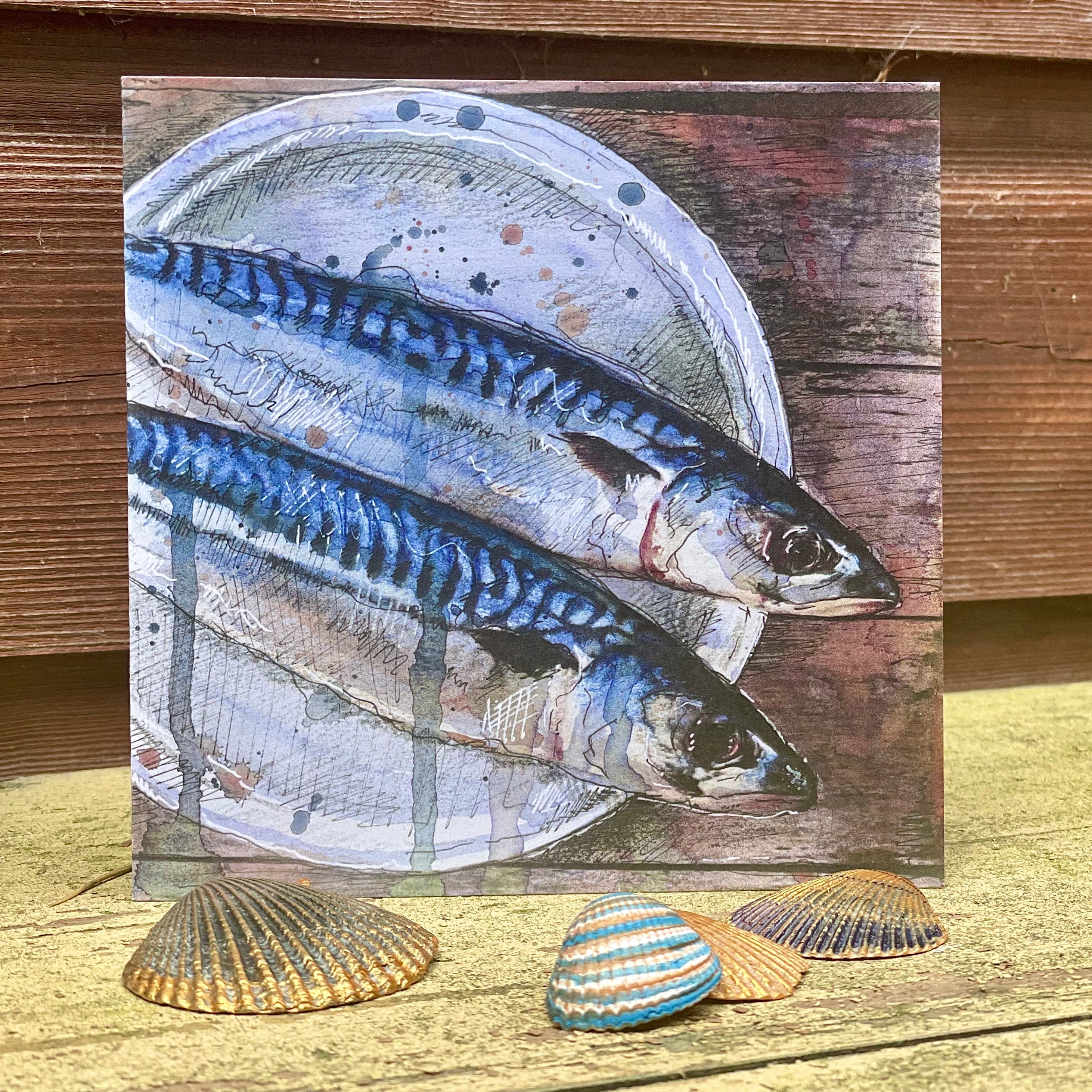The image features a detailed watercolor painting on a small square canvas, showcasing a scene with two bluish-gray, elongated fish, possibly pike, mackerel, or sardines, lying on a white plate. The fish are positioned with one on the bottom and the other slightly above, both angled to the right. The painting depicts a background with a wooden wall, and the canvas itself leans against a lighter-colored, real wooden wall. At the base of the painting, there is an old, worn wooden floor with chipped white paint, revealing a dirty, yellowish hue. In front of the canvas, there are four clamshells arranged as decoration, including a large flat one and a blue, white, and brown striped one. The overall setting suggests an indoor environment with a weathered, rustic aesthetic.